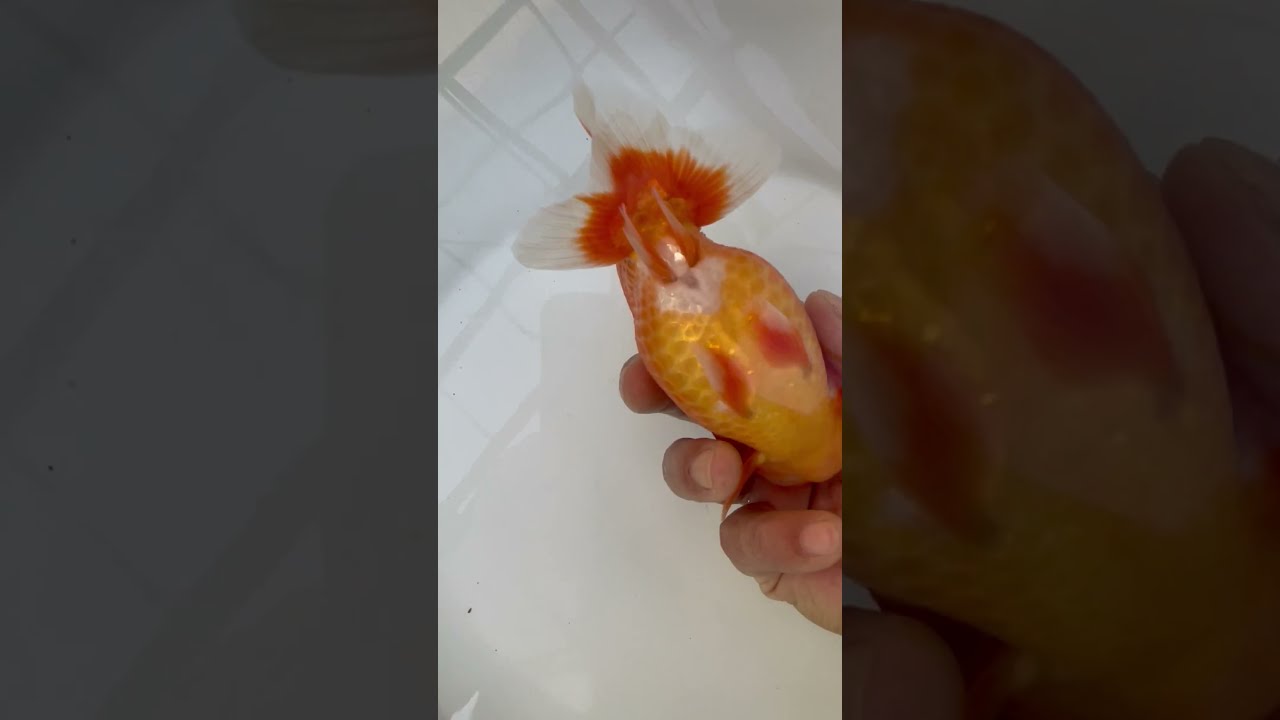In the image, a white hand, possibly male, is seen holding a good-sized goldfish by its head, with the thumb and fingers wrapped around the fish. The goldfish, which has a vibrant orange-gold body and an orange tail, appears lifeless with no visible movement. Behind the goldfish, there is a white background with various shapes and a wide, faded border on the left and right sides, created from the main image. It is suggested that the fish might be held over a toilet or inside a white bucket, hinting at a ceremonial burial for a child's pet. The scene poignantly represents the common end for goldfish, which often have brief lifespans.